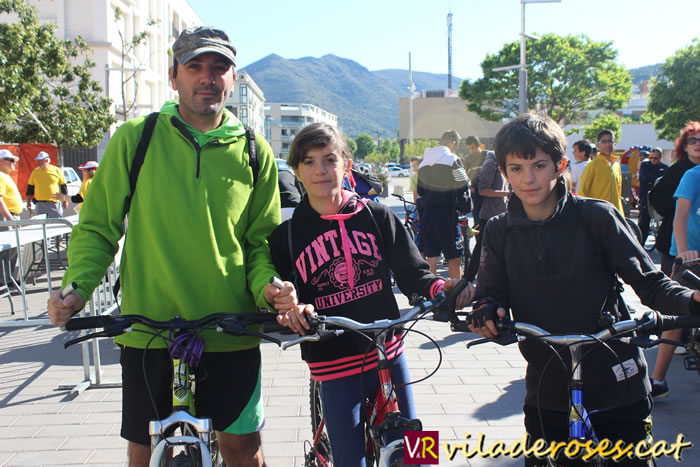The image features a family—comprising a father and two children—posed on bicycles against a scenic backdrop. The father, positioned on the left, is donned in a green sweatshirt, a green shirt underneath, a gray baseball cap, black shorts with green stripes, and a backpack with black straps. He rides a green bicycle with black handlebars and a silver fork. To his right is the daughter, wearing a black sweatshirt with pink lettering that reads "Vintage University" and blue sweatpants, standing next to her red bicycle. Further to the right is the son, outfitted in a black sweatshirt, black pants, and gloves, alongside his blue bicycle. They are situated on a street paved with stone bricks, surrounded by bustling crowds, fellow cyclists, and workers clad in yellow shirts. The background showcases tall buildings, numerous trees, and a majestic mountain under a gray-blue sky.